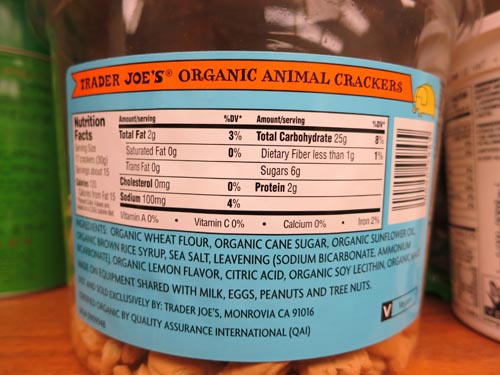A jar of Trader Joe's Organic Animal Crackers is prominently displayed. The jar features a light blue label adorned with an orange ribbon at the top. Bold black text indicates the product name: "Trader Joe's Organic Animal Crackers." To the right of the text is an illustration of a yellow elephant. The jar's lid is made of clear plastic.

At the bottom of the jar, there is a stack of animal-shaped crackers, clearly visible through the transparent container. Below the main label is a detailed Nutrition Facts panel. Key nutritional information includes: serving size details, total fat content of 2 grams, 0 grams of cholesterol, 100 milligrams of sodium, total carbohydrates of 25 grams, and sugars amounting to 6 grams. 

The ingredients list contains organic wheat flour, organic cane sugar, organic sunflower oil, brown rice cereal, sea salt, leavening agents (ammonium bicarbonate), citric acid, and sorghum flour. An allergen warning notes the presence of milk, eggs, peanuts, and tree nuts. The product is distributed by Trader Joe's, located in Monrovia, California.